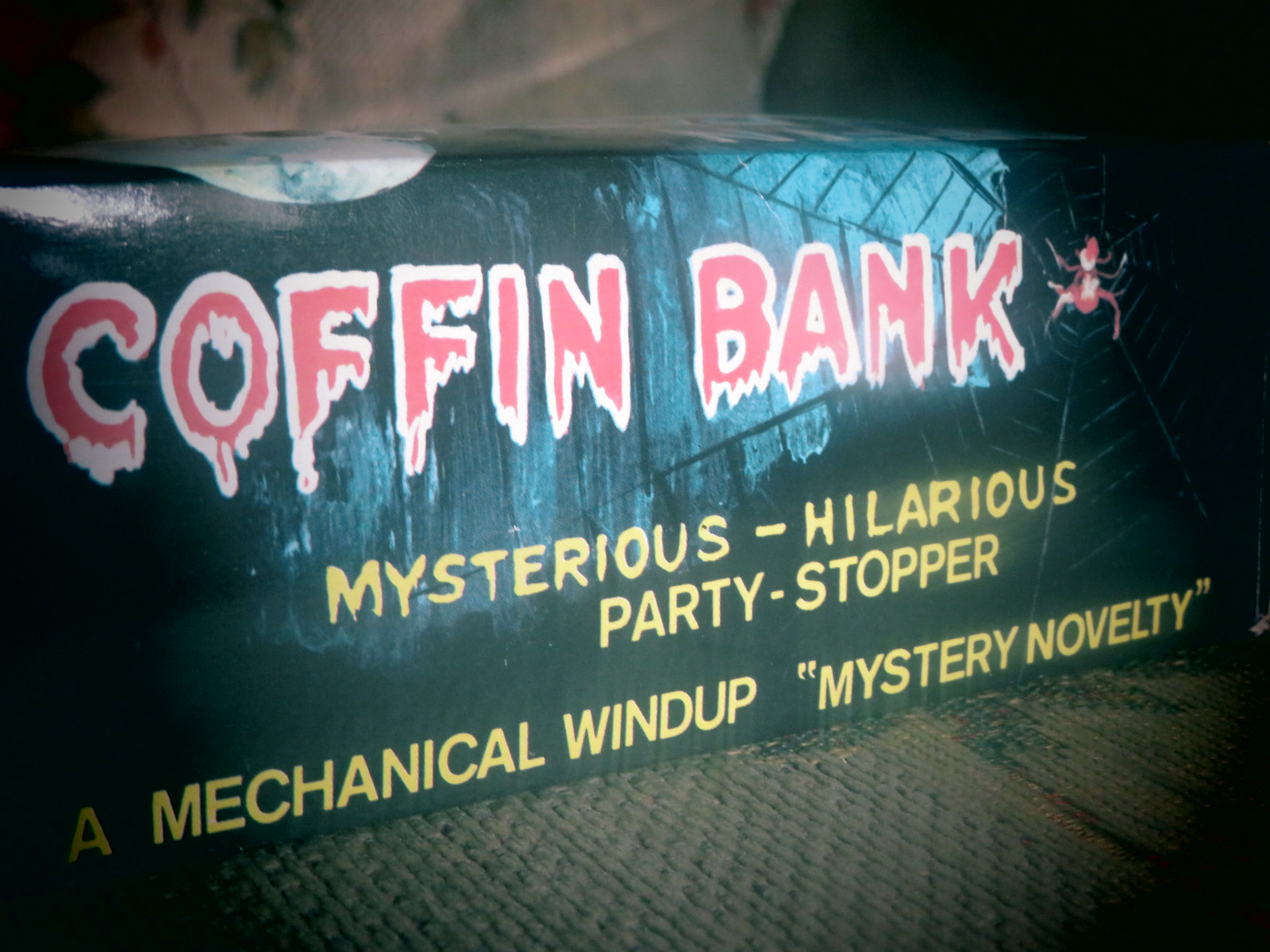The image depicts a digitally created, long rectangular black box situated on a fabric material, most likely at night. In the upper right-hand corner, a spider web extends from a red spider, seemingly illuminated by a moonlit backdrop. At the box's center, the words "COFFIN BANK" are prominently displayed in a red font with a white border, designed to appear as if they are dripping, reminiscent of blood. Below this title, in yellow text, are the phrases "MYSTERIOUS-HILARIOUS PARTY-STOPPER," "A MECHANICAL WIND-UP," and "MYSTERY NOVELTY." A partial moon can be seen peeking out from the upper left, adding to the eerie atmosphere.